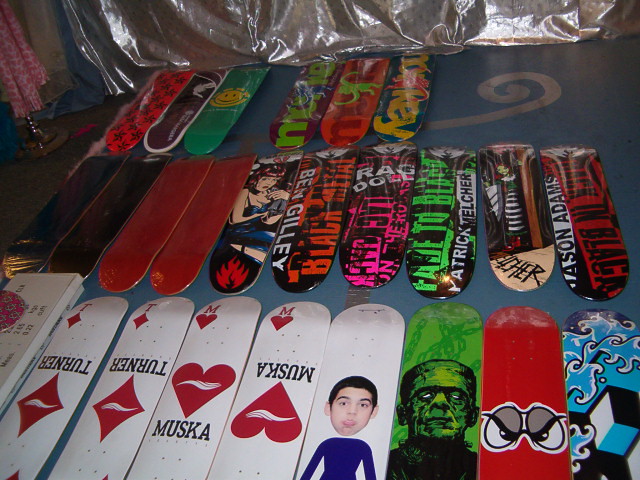This photograph, taken from an overhead angle, displays several finger-sized skateboards without wheels, neatly arranged on a blue surface adorned with silver, swirling lines. The image is divided into three distinct rows.

In the top row, there are six skateboards, each varying in color and graphics. The first is red with black stars, followed by a black skateboard with a white border. Next to it is a green skateboard featuring a yellow smiley face. The remaining three have the word "Monkey" written on them: one is purple with green text, another is orange with red text, and the last is blue with yellow text.

The middle row consists of several skateboards. The first four, positioned from left to right, include two plain black and two plain red ones. The next six skateboards, primarily black with neon lettering, feature various designs. Notably, one of them depicts a woman in a black dress with flames at the bottom. Towards the right end of this row, two stacked skateboards include unidentifiable writing.

The bottom row features seven skateboards. Four are designed to resemble playing cards featuring hearts and the word "Mooska," with one particularly marked with the name "Turner" beside a diamond symbol. Alongside these, there are skateboards with distinct graphics: a green one with Frankenstein, a red one with eyes reminiscent of Angry Birds, and a blue one displaying light bluish waves.

In the background, partially visible, are what appear to be articles of fabric or clothing, enhancing the scene's intriguing composition. Some skateboards remain in their packaging, indicating they are brand new and have yet to be used.